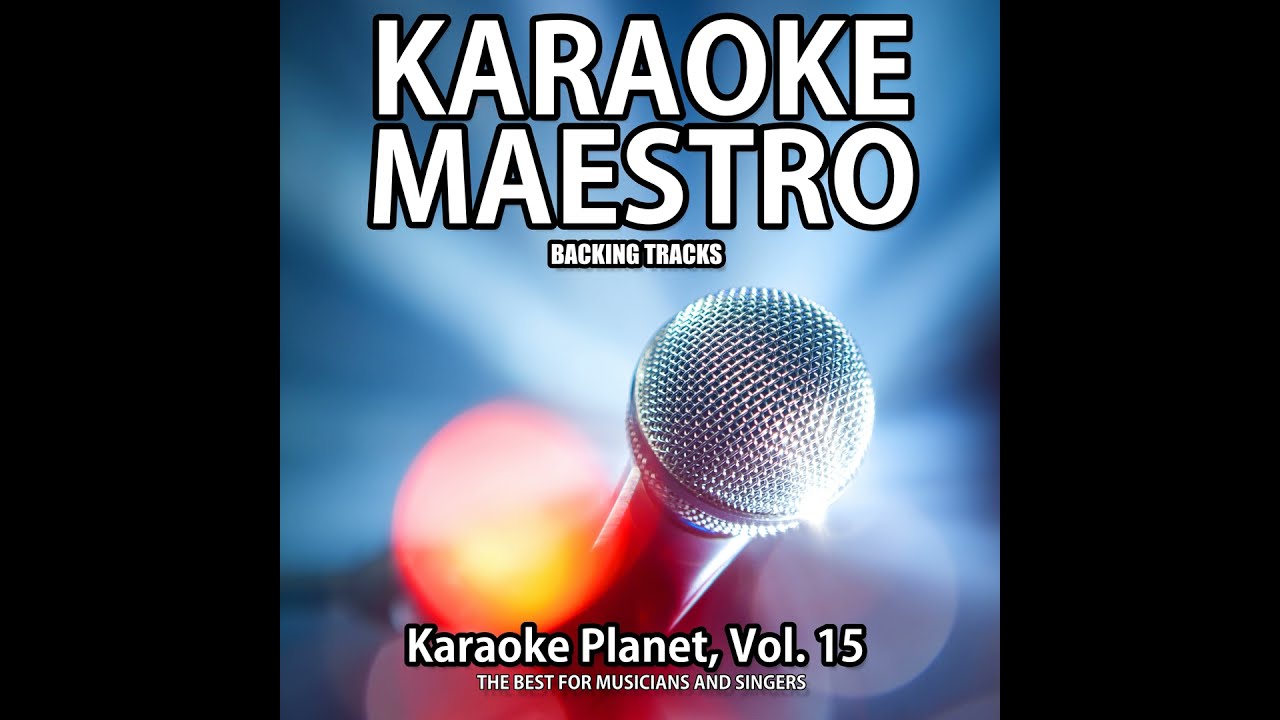The image is a vividly designed poster, predominantly featuring a classic silver-headed, black-bodied microphone at its center. Behind the microphone, there's a bright, shiny light that creates a striking halo effect against a predominantly blue, blurred background adorned with red, amber, and white orbs. The borders of the image are accentuated by two vertical black strips on either side, creating a letterbox effect.

At the top of the poster, in large white capital letters outlined in black, the text reads "Karaoke Maestro". Below this, in smaller white and black-outlined capital letters, it states "backing tracks". At the bottom, again in white letters outlined in black, the text proclaims "Karaoke Planet, Vol. 15", followed by the tagline "the best for musicians and singers". This detailed composition and sophisticated color scheme make the poster visually appealing and suggestive of a CD cover or promotional flyer for a karaoke music collection.